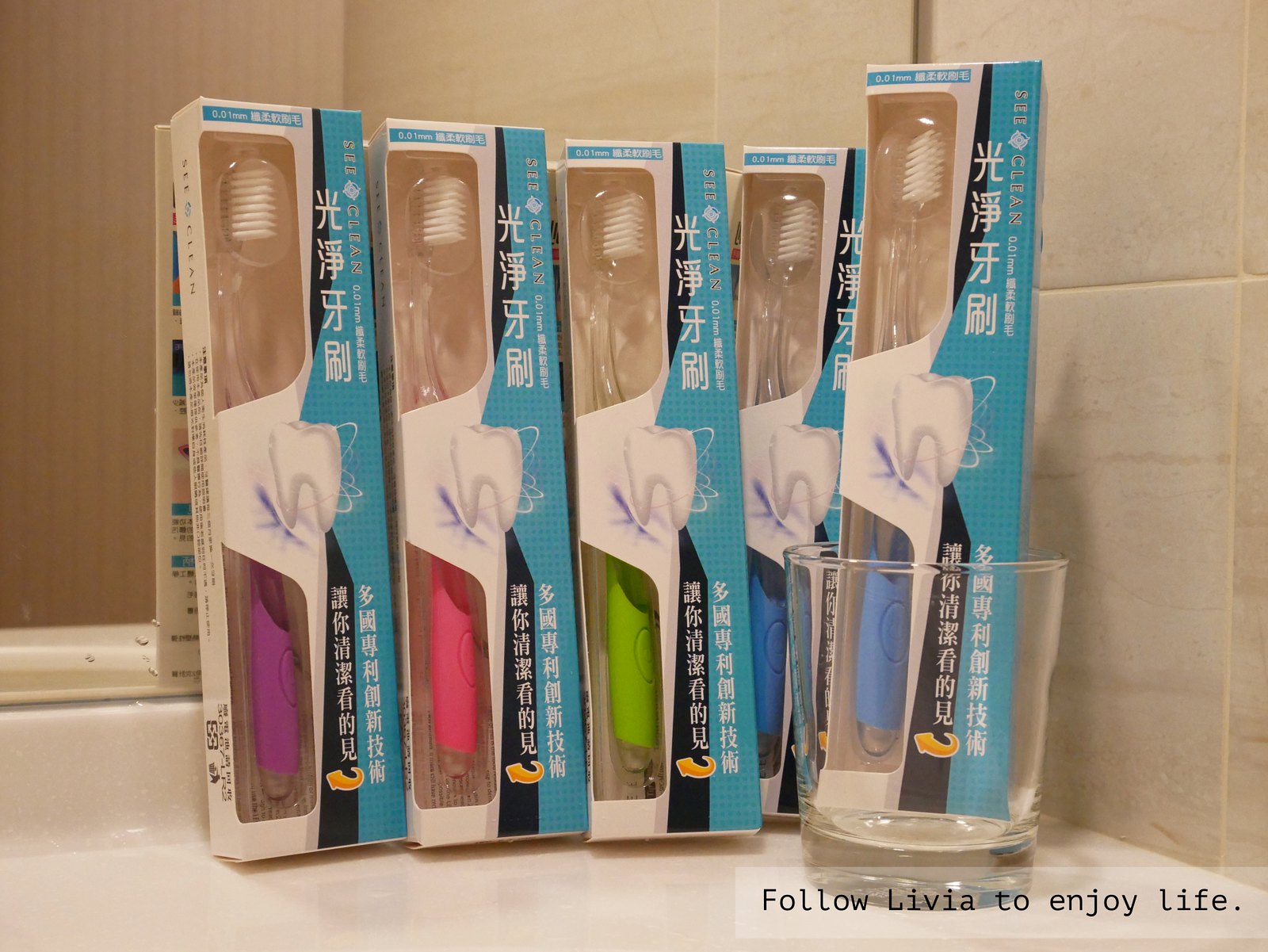This detailed image captures five brand new toothbrushes still sealed in their original blue and white packaging with text written in an Asian language, possibly Chinese. The toothbrushes are displayed on a white bathroom counter accompanied by a mirror, with an off-white, beige-tiled wall with marbling visible to the right. From left to right, the toothbrushes are distinguished by their vibrant handle colors: purple, pink, lime green, dark blue, and light blue. Notably, the light blue toothbrush on the far right is placed inside a clear glass tumbler, making it appear slightly longer. Each package prominently features an image of a tooth encircled by white lines. At the bottom of the image, black text reads, "Follow Livia to enjoy life."